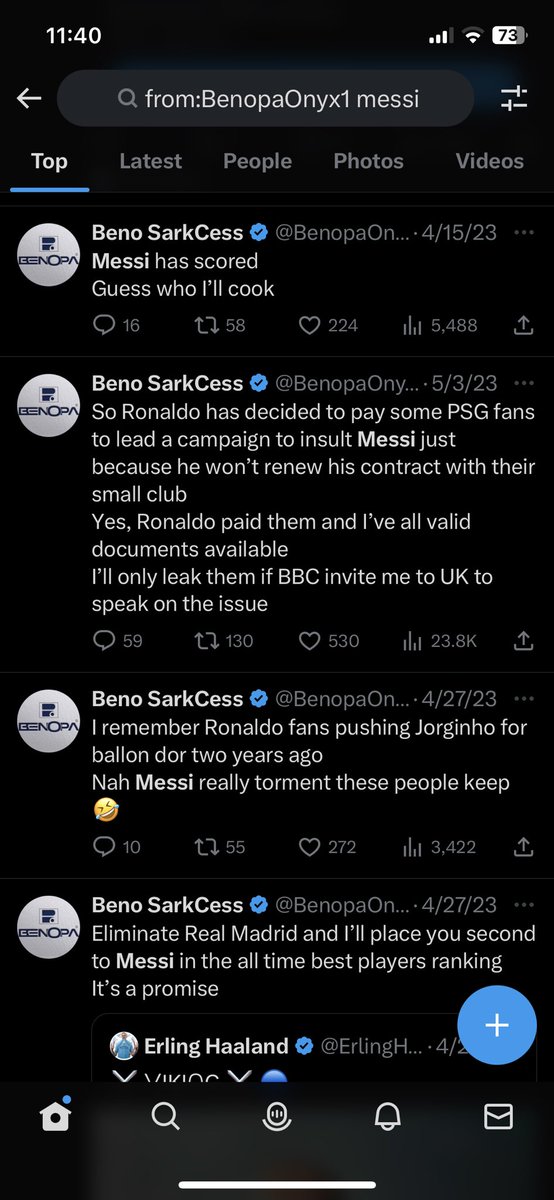A screenshot captured from a cell phone displays a series of comments associated with the name "benopa onyx." At the top of the screenshot, the search bar starts with "from: benopa onyx 1 M-E-S-S-I," though it cuts off. The user's name is also displayed as "beno sarkcess." The visible top comment reads: "Messi has scored. Guess who I'll cook."

Scrolling further, another comment by the same user states: "So, Ronaldo has decided to pay some PSG fans to lead a campaign to insult Messi just because he won't renew his contract with their small club. Yes, Ronaldo paid them, and I've all valid documents available. I'll only leak them if BBC invites me to the UK to speak on the issue."

As the screenshot continues, another comment from "beno sarkcess" emerges: "I remember Ronaldo fans pushing for Jorginho for Ballon d'Or two years ago. Nah, Messi really torments these people, keep," followed by a laughing face emoji.

The final visible comment by the same user declares: "Eliminate Real Madrid, and I'll place you second to Messi in the all-time best players ranking, it's a promise."